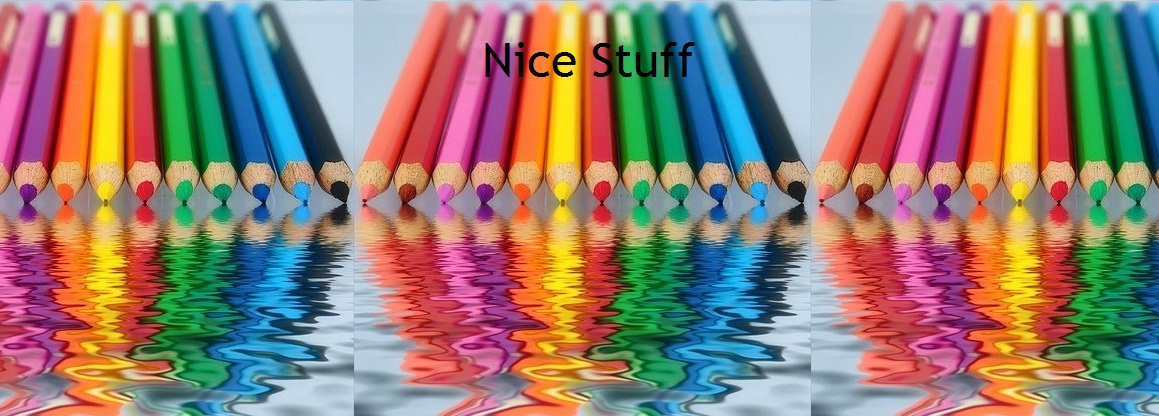This color photograph displays three sets of colored pencils arranged across the top portion of the image. Each set contains 12 colored pencils, which extend beyond the image's boundaries at the left and right edges, while the middle set is fully visible. The vibrant pencils include colors like pink, red, purple, yellow, orange, green, blue, black, and the natural tan of the wood. They are meticulously sharpened and point towards the camera. 

A notable feature in the image is the mirrored reflection of the pencils in a pool of water occupying the lower part of the composition, reinforcing their vivid colors. 

The background is a light blue, enhancing the contrast and sharpness of the pencils. Centered above the middle set of pencils, bold black text reads "NICE STUFF," adding a striking textual element to the photograph.